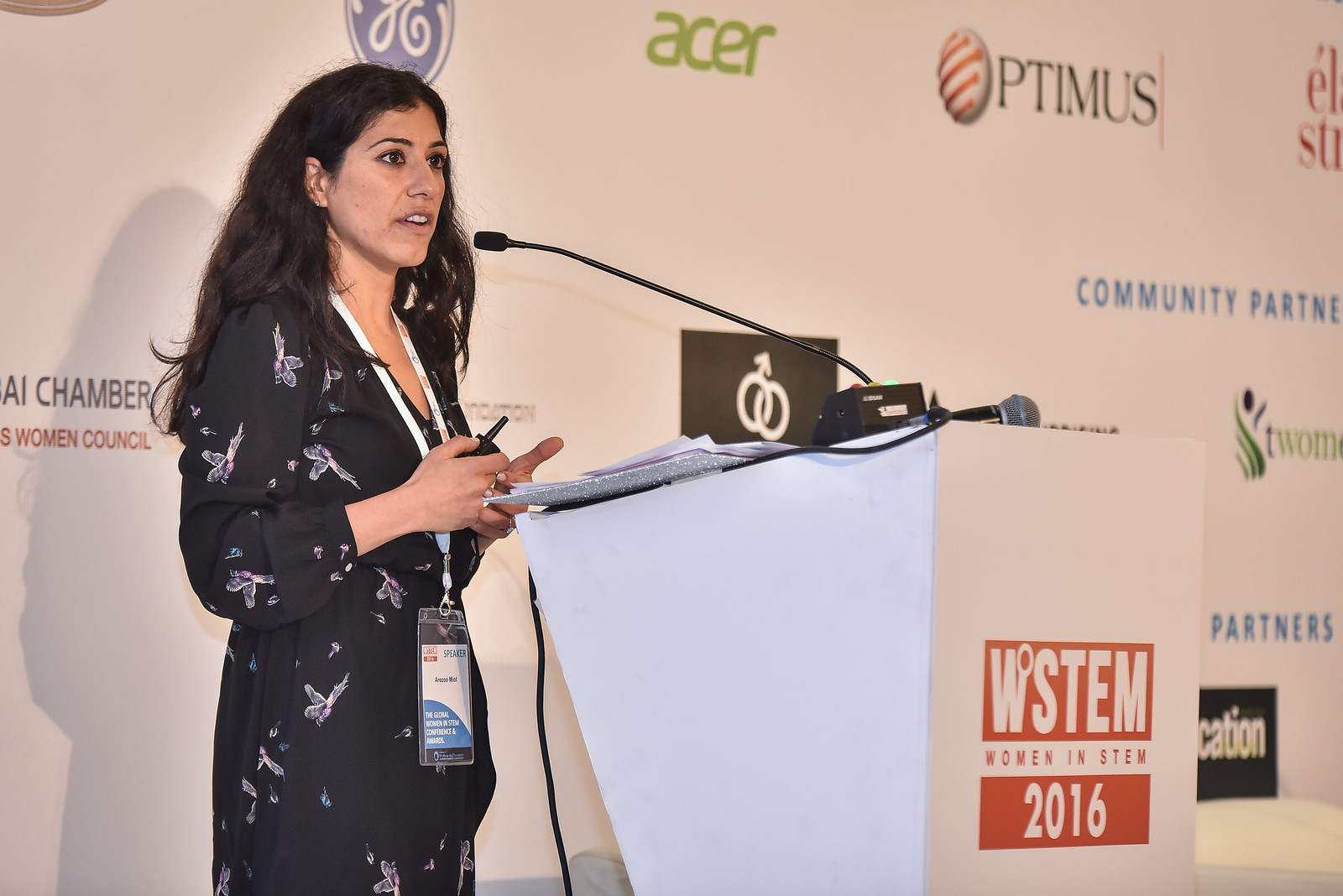In this image, a woman with long black hair is speaking at a podium during the Global Women in STEM Conference and Awards. She is wearing a black dress adorned with butterflies and has a white lanyard with a name tag around her neck. The white podium features two red rectangles; the upper one contains the text "WSTEM" in white and "Women in STEM" in red, while the lower one reads "2016" in white text. A microphone is positioned towards her as she addresses the audience. Behind her, the backdrop is filled with various brand logos, including GE, General Electric, Acer, P. Timmis, and Optimus. The overall setting suggests a formal event aimed at celebrating women's contributions to the STEM fields.